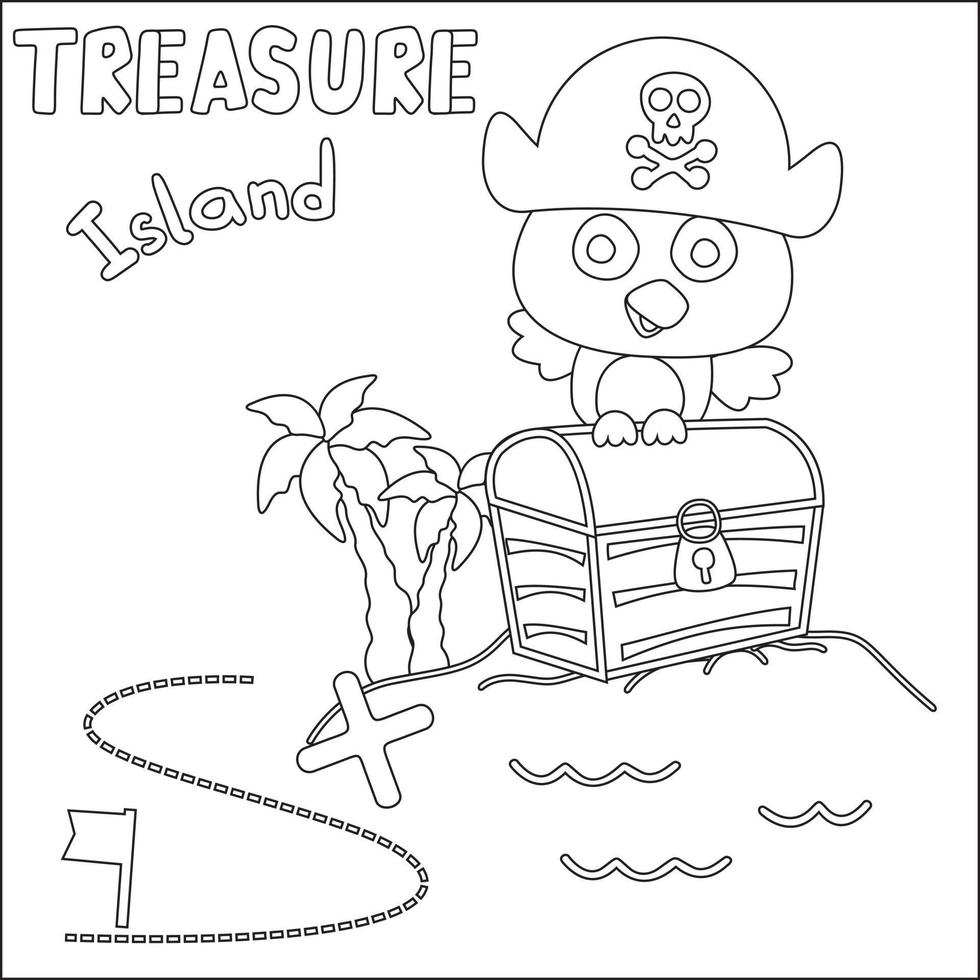This illustration is a detailed black-and-white line drawing that prominently features the title "Treasure Island" at the top left corner. The image centers around a playful, comic-style scene set on a small island. Atop a treasure chest, which has a lock on its front, sits a pirate owl or a parrot, distinguished by its pirate hat adorned with a skull and crossbones. The bird, looking directly at the viewer, raises its wings in the air. The island is flanked by two palm trees, and underneath one of the trees lies an X marking the spot. A dotted line meanders from this X and leads to a flag blowing towards the left in the bottom left corner of the image. The entire illustration, with its simple yet charming details, resembles a page from a child's coloring book, inviting young artists to bring it to life with color.